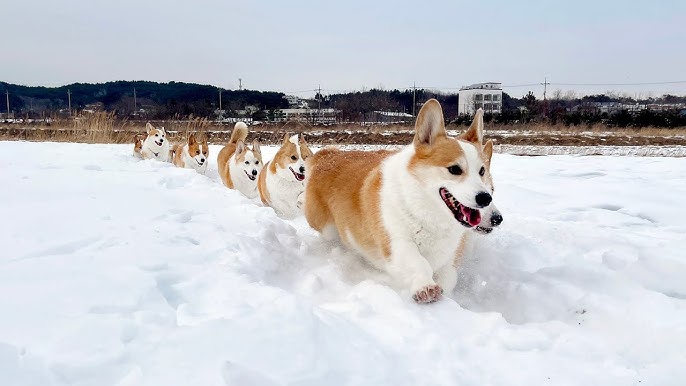The photograph, likely taken outdoors, captures an energetic group of approximately eight corgis sprinting through pristine white snow in a straight line. The corgis, identifiable by their short legs, big ears, and elongated bodies, exhibit distinctive white faces and upper bodies contrasted by light brown or beige fur. Their joyful expressions, with mouths turned upward, reflect their excitement and energy as they plow through the snow at high speeds. The snow is noticeably less deep along the path they've carved, with thicker snow flanking both sides. In the background, a landscape of weed-covered grounds is visible, leading into a distant view of tree-covered mountains dotted with buildings and intersected by power lines. The overcast sky above adds a grayish hue to the scene, which might give the impression of digital manipulation, though the natural charm of the scene remains intact. This lively depiction of corgis enjoying their sprint through the snow is both captivating and heartwarming.